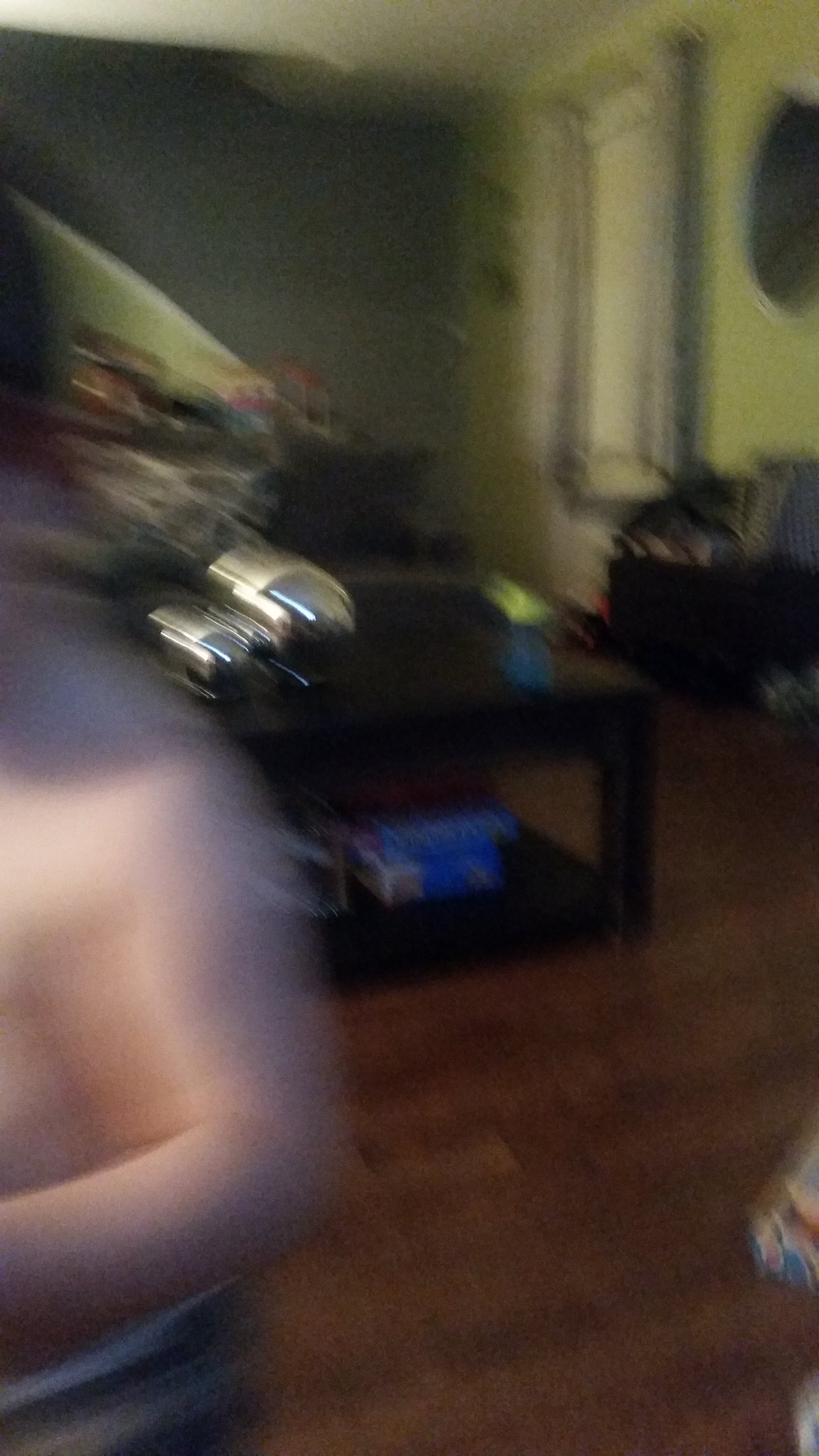This highly blurred photograph captures the corner of a room inside a home, merging multiple visual elements into a hazy, almost dreamlike composition. On the left side, there is the indistinct form of a shirtless figure, seemingly in motion, revealing a bare arm, shoulder, and part of the ribcage, potentially with some metallic objects or bullets on or near the shoulder. The central focus of the image is a black square table, notable for its stark presence amidst the blur. On the tabletop, barely visible, are a yellow rectangle and a blue rectangle, their identities uncertain due to the blur. Beneath the table, a shelf holds two blue packages that might be printer paper. The floor is a dark wood, possibly laminate or pressed vinyl, exhibiting a brown hue with hints of red. In the background, to the right, there seems to be a long narrow window or mirror next to an indeterminate piece of furniture. The room's walls transition from a light color to a dark shade, with a white ceiling capping the scene.